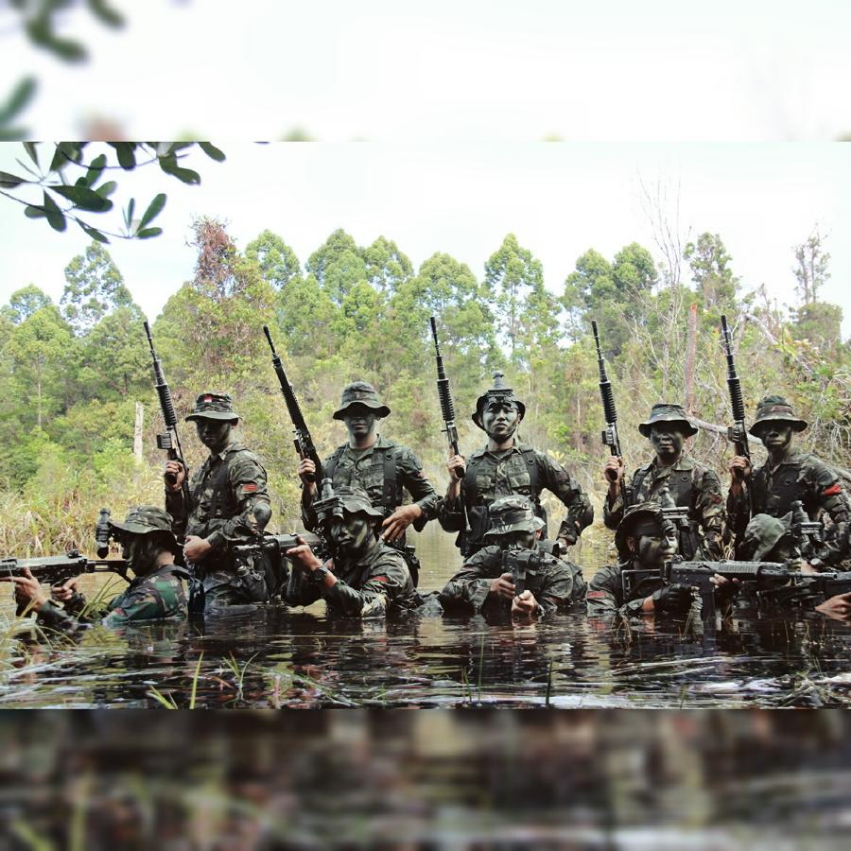The image captures a group of soldiers poised for a photograph in a swampy environment. It is a vertical, rectangular picture with a light blue, slightly overcast sky. The background features a dense tree line with various shades of green and some brown and white stems. Tall, light green grass dominates the scene, and a murky, brown, pond-like swamp with patches of green growth surrounds the soldiers.

The soldiers are organized in two distinct rows within the swamp. The front row has soldiers in a crouching position with the dark, murky water reaching up to their shoulders. Each soldier in this row is aiming their black and silver rifles in various directions. The back row shows soldiers standing with the water up to their waists, holding their rifles pointed skyward. All soldiers are dressed in dark green camouflage outfits and cloth caps, with their faces painted in dark green camo. Some soldiers have night vision goggles mounted on their caps.

This scene gives off a strategic and tactical vibe, capturing the soldiers—who appear to be from a foreign military force or possibly special operations without clear U.S. markings.